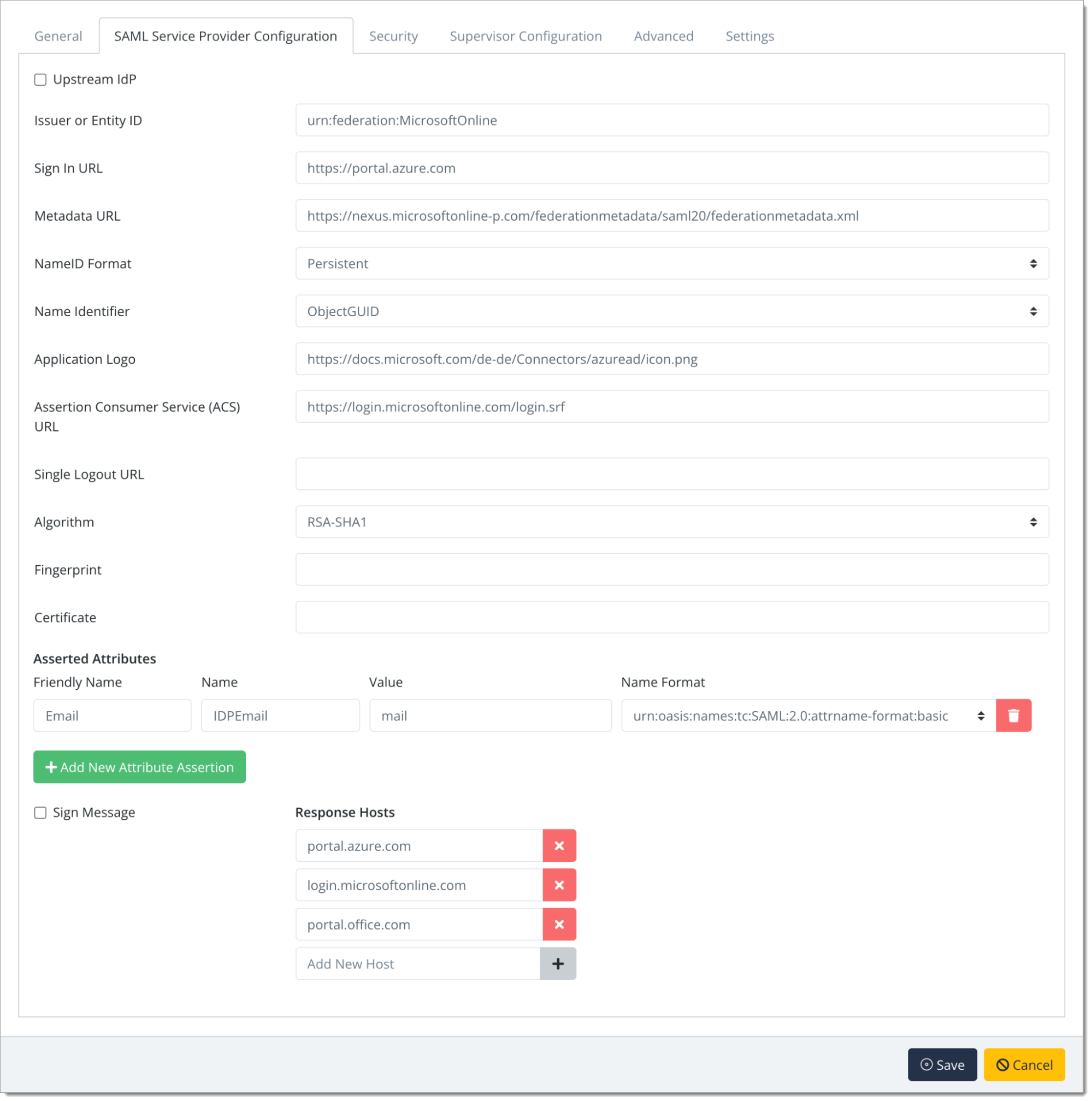A screenshot of a technical configuration page for SAML (Security Assertion Markup Language) settings within a network or site management interface. At the top, there are multiple tabs visible, including General, SAML, Service Provider, Configuration, Security, Supervisor, Advanced, and Settings. The focus is on the SAML section, displaying a series of fields and options for setup. Users can input details or select from dropdown menus for fields such as Issuer, Entity ID, Sign-in URL, Metadata URL, Name ID Format, Name Identifier, Fingerprint, Certificate, and Algorithm, with the latter showing RSA-SHA1. Additionally, there are areas for configuring Asserted Attributes, requiring a friendly name, name value, and name format, with an option to select Signed Message. Further down, the page features settings for Response Hosts, containing several URLs associated with Microsoft services. The interface is designed for advanced users familiar with network security and SAML configurations.